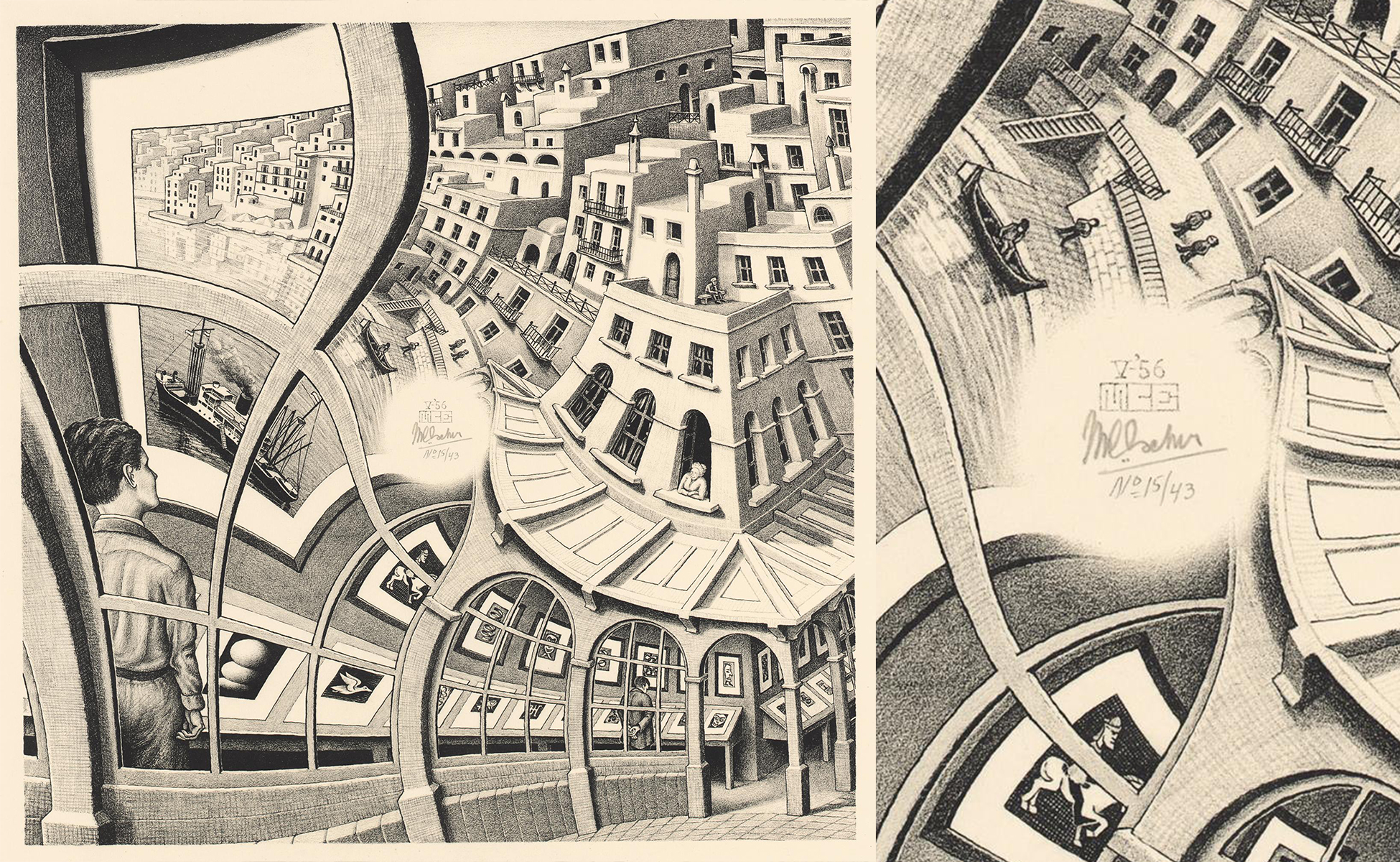The image is a detailed black and white print composed of two sketches side by side. Done in either pencil, charcoal, or a similar medium, the leftmost sketch portrays an abstract hallway scene with a man visible through an arched window. He is gazing at paintings on a wall that seamlessly blend into the hallway’s roof, creating an illusion where the depicted cityscape of blocky buildings merges with the architectural space. In the top left corner of the left sketch, a steamboat and dock area add to the surreal atmosphere.

On the right, a continuation from a different angle showcases a similarly abstract and distorted urban environment. Various rowboats and buildings with metal balconies and bent window frames are depicted, reflecting the same blending effect as the left image, where paintings morph into the hallways. The consistent curvature and stretching of buildings across both sketches contribute to a coherent yet dreamlike cityscape.